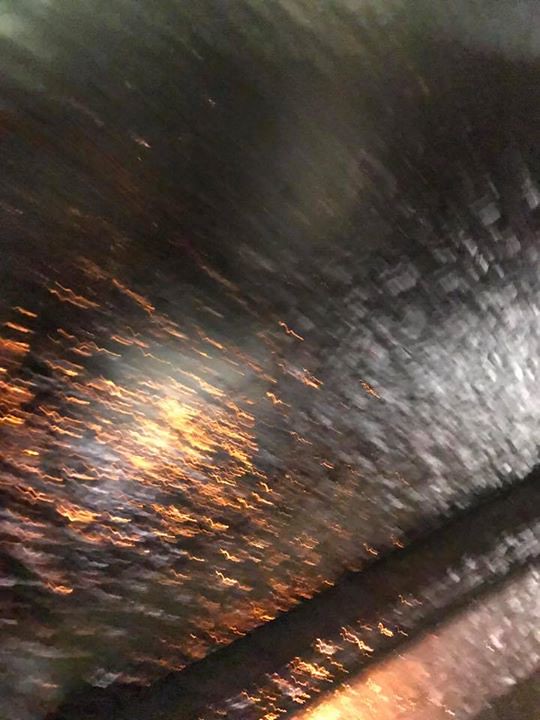A very blurry and abstract image appears, showcasing a predominantly dark scene with no clear subject. The texture and shading suggest it might be a close-up of a wet pavement or an oil slick, reflecting dim ambient lighting. In the bottom right corner, a series of lines are faintly visible, possibly indicating street markings or cracks in the surface. An orange and red reflection, resembling car headlights, adds a splash of color amidst the gloom. The top section remains enveloped in deep shadow, while the lower parts gradually lighten, though still lacking in distinct, identifiable features. The image's ambiguity leaves much to the imagination, evoking an eerie and mysterious atmosphere.